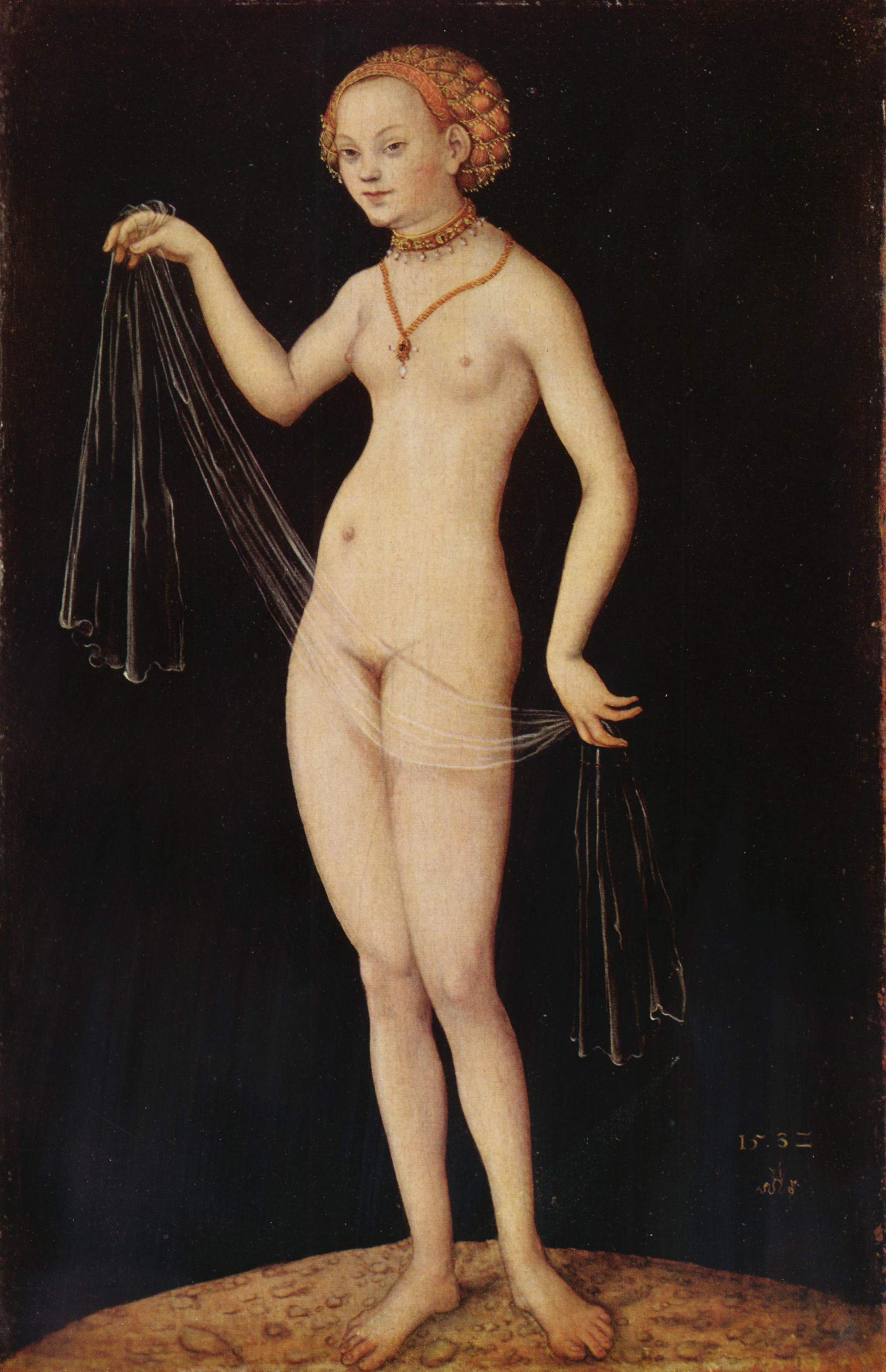The painting depicts a young, nude woman standing on a beige circular pedestal, holding a diaphanous, see-through scarf in both hands, which accentuates her thin figure. Her red-blonde hair is styled in a bun, intricately held together by a beaded net. She wears two striking necklaces: an expensive one with beads hanging from the edges and a choker around her neck. Her small breasts and pale white skin contrast with the dark, almost black background, which features an indistinct signature and a date from the 16th century in the lower right corner. The overall tone is a rich mix of brown, black, and a hint of gold. She gazes off to the left, adding a contemplative air to her poised stance on what appears to be a chalky, earthy patch.